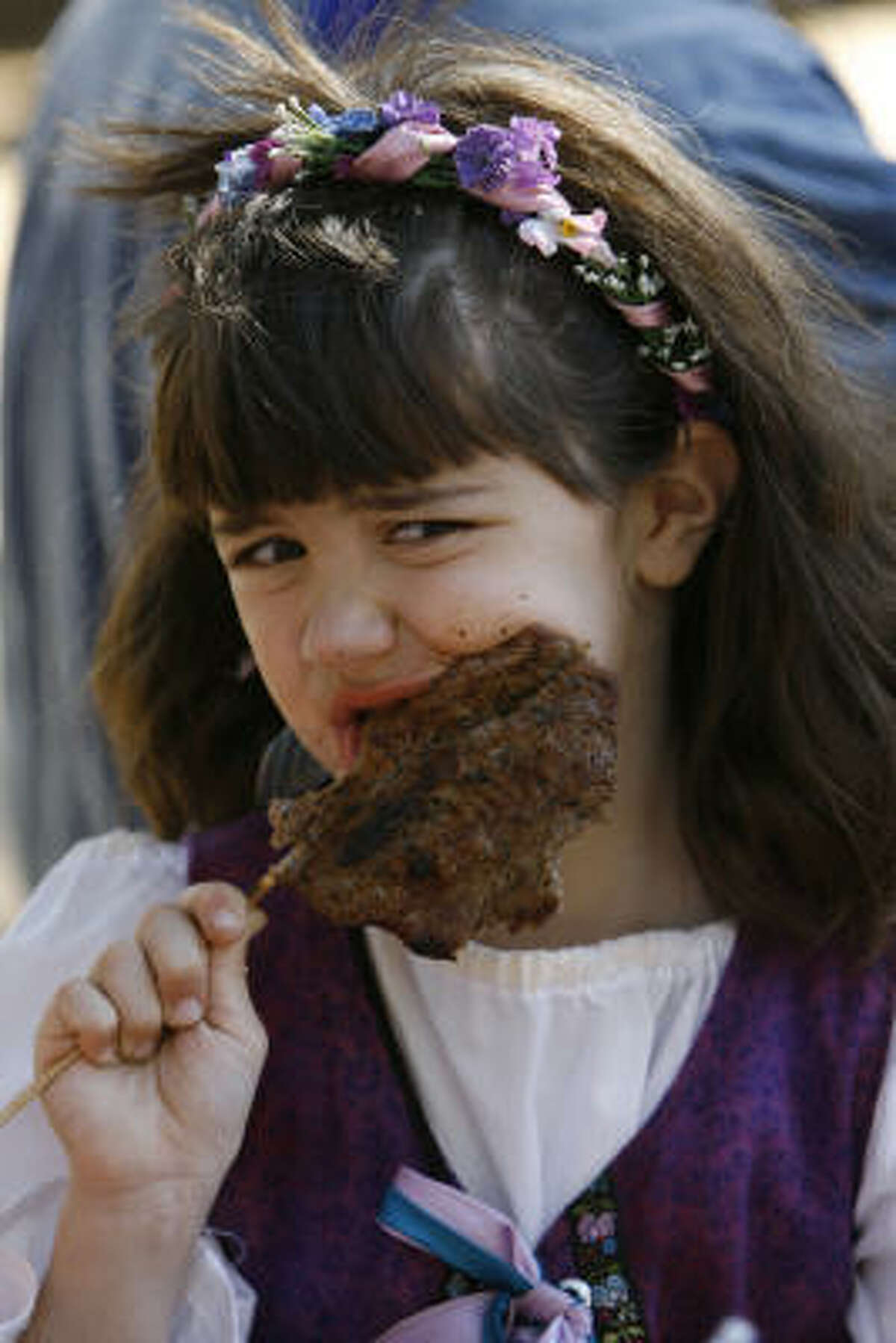The photograph features a young girl, approximately ten years old, who is caught mid-bite while eating meat on a stick. She occupies the central portion of the image, visible from her chest upwards, and the background is blurred, suggesting an outdoor setting like a barbecue. The girl is dressed in a traditional-style outfit: a purple vest fastened with a lilac silk ribbon over a white shirt with frilly sleeves ending at her forearms. Her brown hair is adorned with a floral headband wrapped in a pink ribbon. She has a slightly worried expression as she bites into the meat, with specks of meat and sauce on her cheek, and she gazes to the right while her body faces forward.